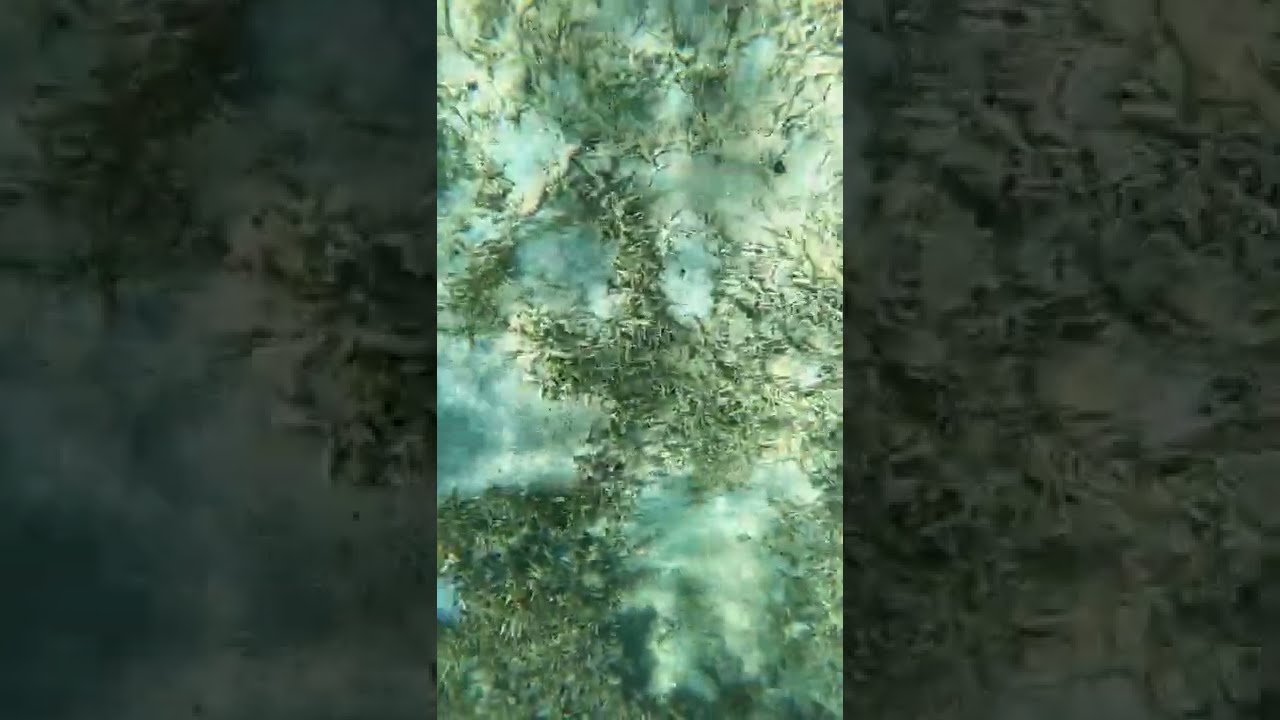The image is an abstract, low-resolution scene that could be interpreted as either a photograph or a digitally generated artwork. It is divided into three vertical sections. The central third of the image features a green, grass-like pattern interspersed with lighter blue-green, cloud-like shapes that give an appearance of dappled patches, reminiscent of moss or algae growing on water. The right and left thirds of the image present a magnified and darkened version of the same pattern, obscuring the green hues and rendering the shapes as shadowy forms. The central pattern is detailed enough to evoke comparisons to a microscopic shot of a bacterial sample, with green elements that resemble pine needles or voodoo dolls laid on a foggy forest floor. The overall composition creates a complex, layered scene that blends natural and microscopic imagery.